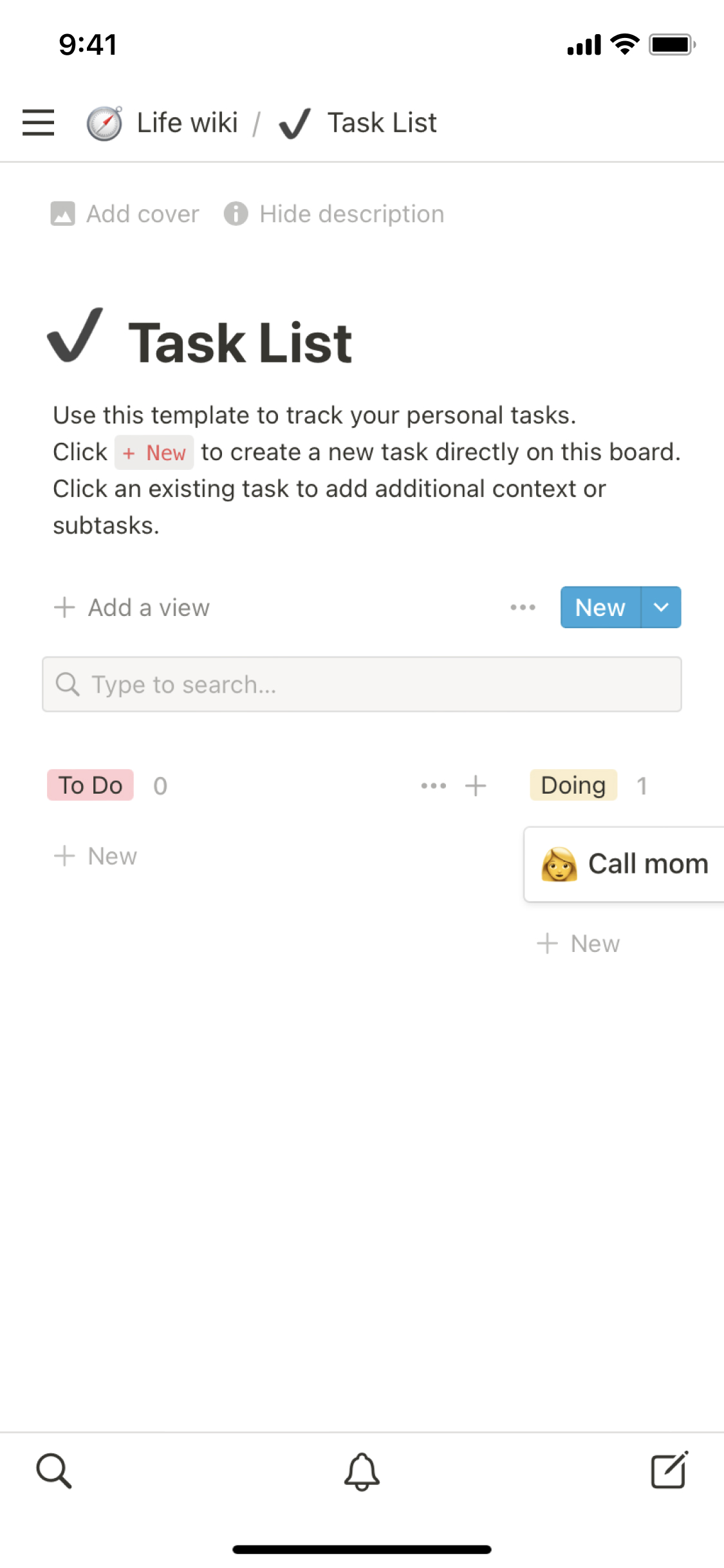This image appears to be a screenshot taken from someone's device, possibly from a productivity application or task management tool. The main focus is on a digital board titled "Life Wiki" or "White Wiki" with a "Task List" section. 

At the top, there is a notable task item with a black checkmark next to it, indicating its completion. Following this, the instructions "Use this template to track your personal tasks" are clearly visible. Underneath, within a gray rectangle, the phrase "Click + New" is printed in red, guiding users to create a new task directly on the board. Additional directions suggest that clicking on an existing task allows one to add further context or subtext.

Below this section, there is a prompt to "Add a View" on the left. To the right, a blue rectangular button labeled "New" in white print provides users with the option to add new elements. Below these options, there's a search bar placeholder reading "type to search..." indicating a search function.

Further down, there are categorized sections for tasks. In the "To Do" section, highlighted in pink, the command "+ New" is visible, suggesting the user add new tasks. In the "Doing" section, a current task titled "Call Mom" is listed alongside an icon of a woman. This area also includes a "+ New" command for adding further entries.

The overall layout and color-coded sections help users visually organize and manage their tasks effectively.